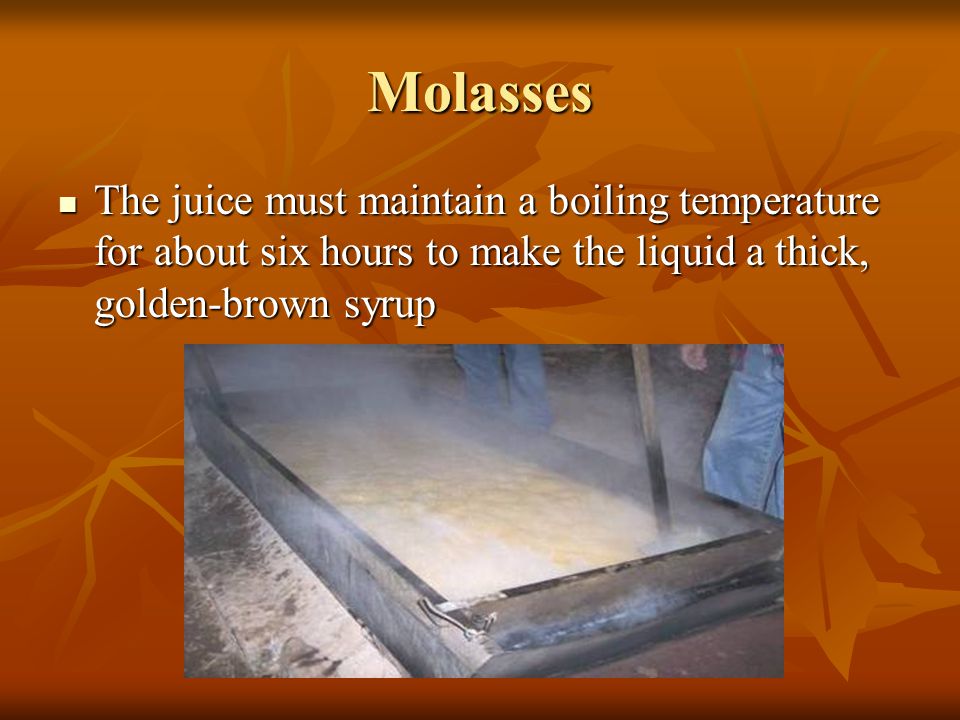The image is titled "Molasses" in yellow Times New Roman font, positioned against a gradient orange background that lightens from a dark, rusty orange at the bottom to a lighter shade at the top. Orange leaves decorate the background, enhancing the earthy tone of the setting. Directly beneath the title, a square bullet point introduces white Times New Roman text explaining, "The juice must maintain a boiling temperature for about six hours to make the liquid a thick, golden brown syrup."

Centered in the image is a photograph showcasing a gray vat filled with boiling molasses. The bubbling, foamy liquid inside the vat emits a white or yellow foam at the top, indicating it is simmering intensely. Surrounding the vat, a couple of individuals, identifiable by their blue jeans, are engaged in the process, each holding a wooden pole to stir the molasses. This scene, depicting hands-on labor, suggests an industrial or work environment dedicated to the process of crafting syrup.